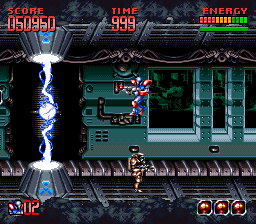This image is a small square screenshot from a video game set in a futuristic laboratory environment. At the center of the screen, two characters are depicted: one is hovering above the other, who stands on a metallic platform. To the left of these characters, a lightning-like laser beam, with swirling blue and white colors, connects the base of the lab to its upper section. In the top left corner, the score is prominently displayed in red. At the top center, a timer shows that 9.99 minutes have been played. The top right corner indicates the energy status. In the bottom left corner, it is shown that the player has two lives remaining. In the bottom right corner, there are three small boxes, likely representing available power-ups or abilities.